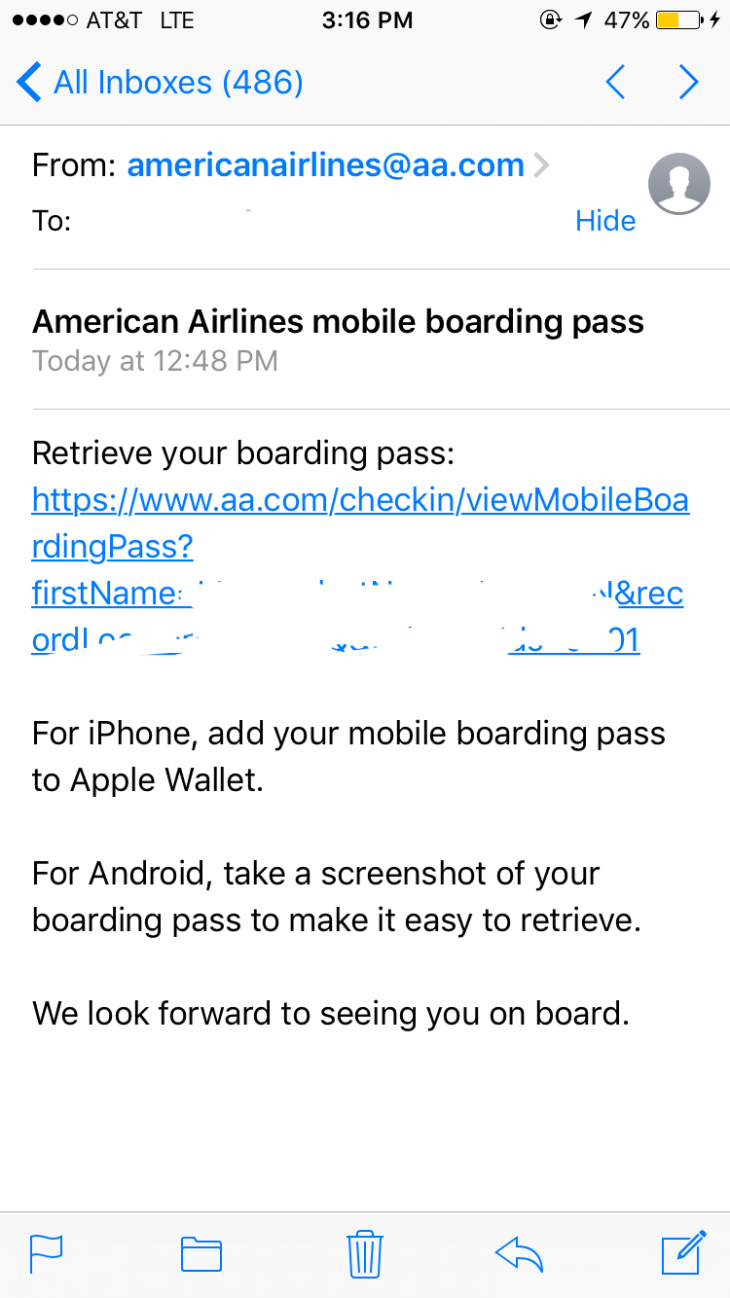The image is a portrait-oriented screenshot of an iPhone's Mail app. In the upper left corner, there are five status indicator circles: four black and one interior white. The status bar reveals an AT&T LTE connection and shows the time as 3:16 PM. On the upper right, icons display the battery level at 47%. 

Below, there's a back arrow indicating a return to "All Inboxes," with a count of 486 emails. Further right, there are left and right navigation arrows. The email snapshot shows a message from American Airlines (email address: aa.com). Although part of the recipient's address is obscured, the subject line reads "American Airlines Mobile Boarding Pass." The email was received today at 12:48 PM.

The email body includes a link (partially omitted) for retrieving the boarding pass and provides instructions for adding it to an Apple Wallet on iPhones or taking a screenshot for Android users. It ends with a statement looking forward to the user's flight and various icons at the bottom of the email.